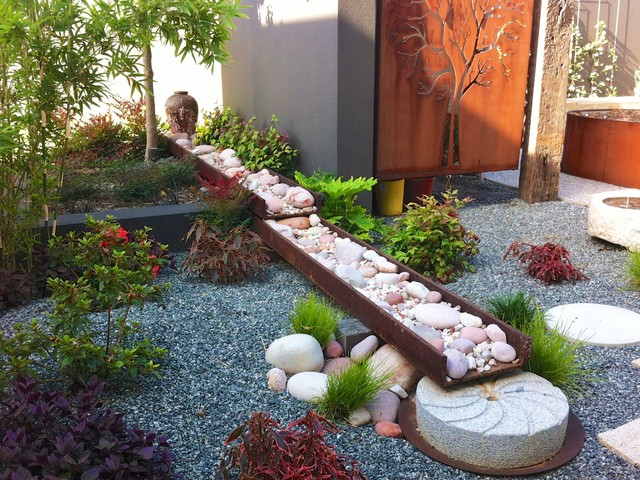This horizontal color photograph captures a tranquil, Asian-inspired zen garden blending elements of both indoor and outdoor aesthetics. The garden features a bed of gray gravel mulch interspersed with various small, mounded plants in shades of green, red, and purple. A prominent feature is a rust-colored metal trough filled with white stones, ranging from pebbles to larger rocks, that cuts diagonally across the image from the back left to the front right. At the end of the trough sits an urn-like vessel, hinting at a water feature.

In the garden's corner, to the right, stands a raised section planted with trees and adorned with a burnt orange basin, which might be holding water or additional plants. A mix of river rocks and mulch adds texture and complexity. The garden is framed by a concrete wall on one side and a bronzed metal gate on the other, with an intricate, skeletal tree design carved into the metal. Hanging trellises add a vertical element to the composition, enhancing the serene atmosphere of this peaceful sanctuary. Above the metal gate, a medium-colored wooden door with a carved tree image beckons from the background, adding a touch of rustic charm to this harmonious outdoor retreat.